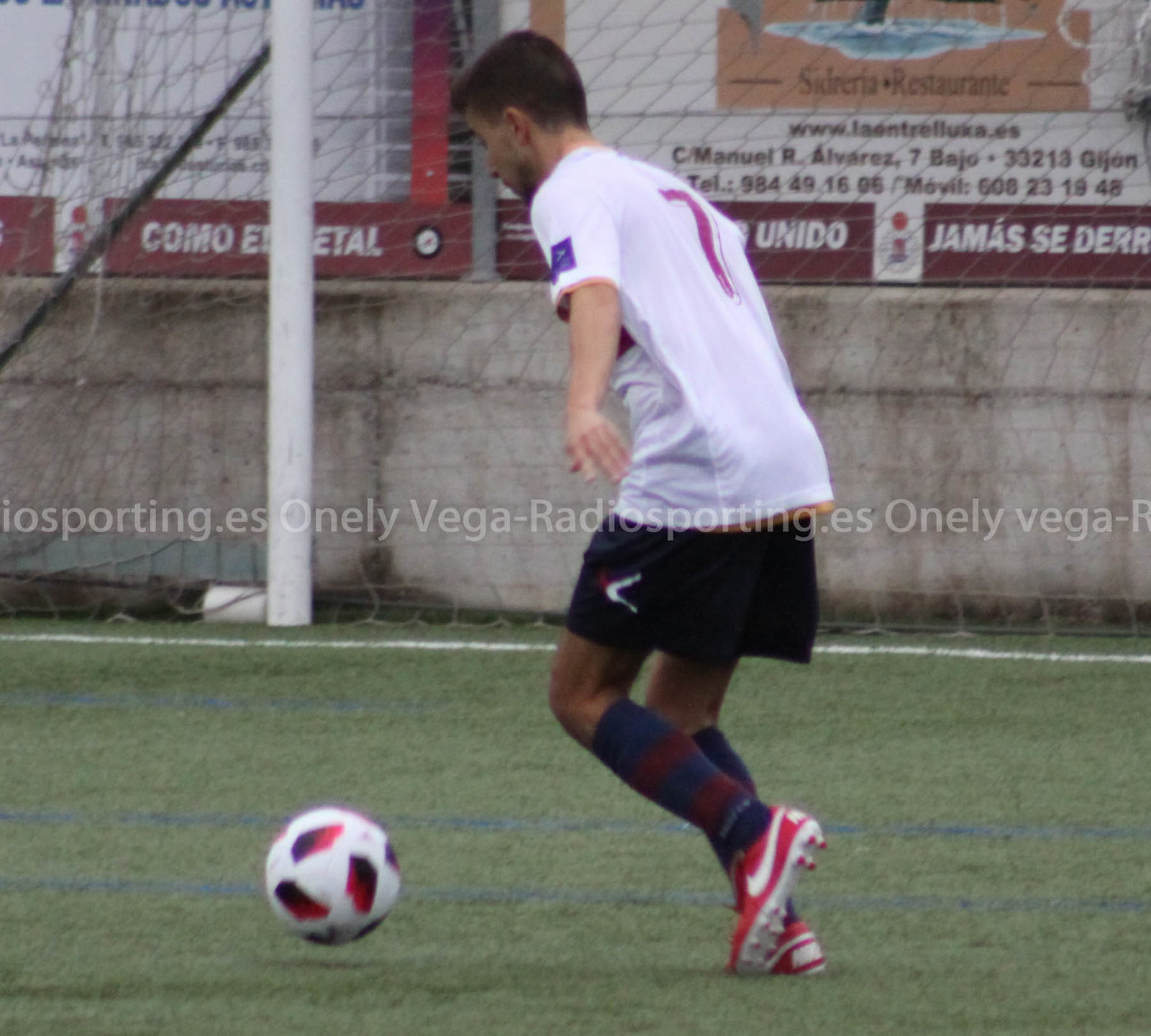This photograph captures a dynamic moment of a soccer player in motion, intensely chasing after a soccer ball on a field covered with vibrant green grass. The player is wearing a white jersey with a red number 7 on the back, black shorts, and red Nike cleats. His socks are navy blue with burgundy stripes, stretching up to meet the hem of his shorts. The player's left arm is extended away from his body as he runs, eyes locked onto the ball just ahead of him, which is predominantly white with black and red swirling designs. 

In the immediate background, slightly to the right of the player, stands the goal, visible with its netting and one of the supporting posts. Beyond the goal, the field is bordered by a metallic fence, and further back, various advertisement boards can be seen. Dominating the center of the image is a horizontal watermark that reads "Vega RadioSporting.es," repeated in a way that simulates a rolling banner.